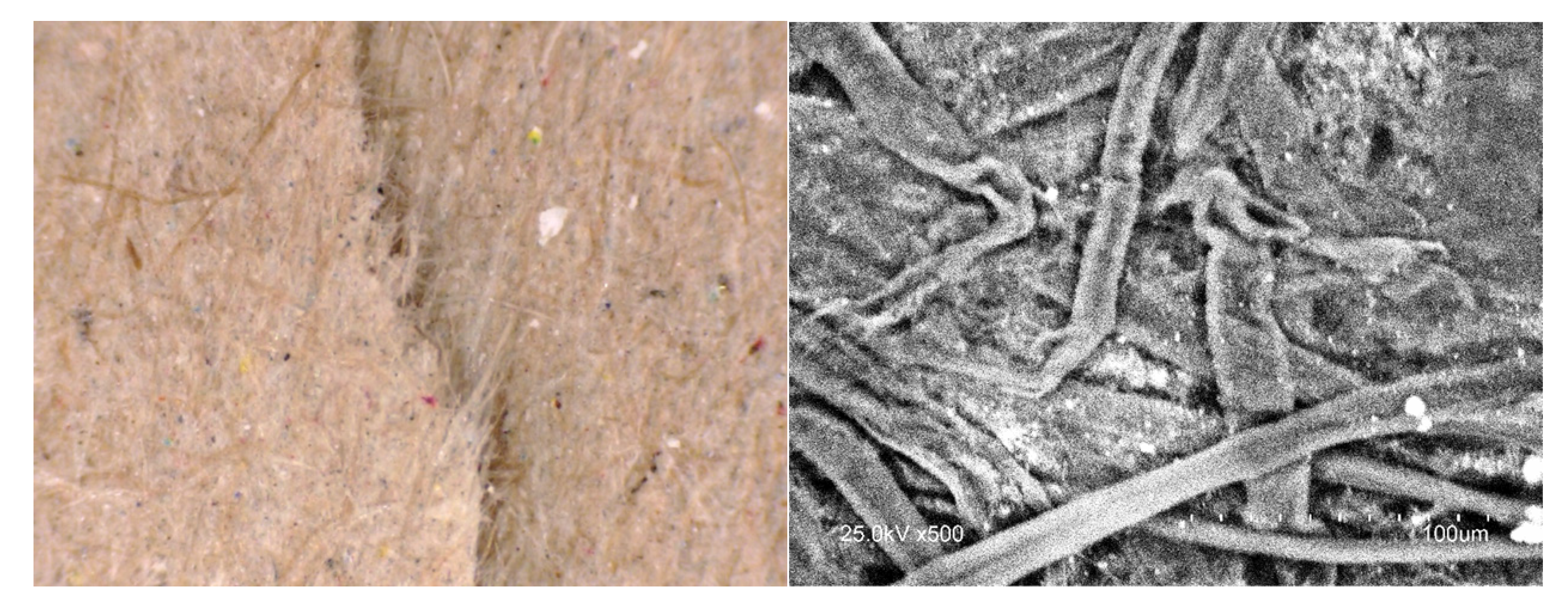The image is a scientific comparison display with two panels side by side. The left panel features a close-up, possibly microscopic, showing a predominantly light brown texture with shades of beige, small red speckles, and finer strands that may suggest dried grass, cardboard fibers, or even animal skin with fur. Meanwhile, the right panel presents a black and white microscopic view with various intersecting strips or strings overlaid on one another, annotated with white text that reads "25.0 kV x 500" at the bottom and "100 µm" towards the right. The overall impression is of detailed, magnified material studies commonly seen in laboratory settings.